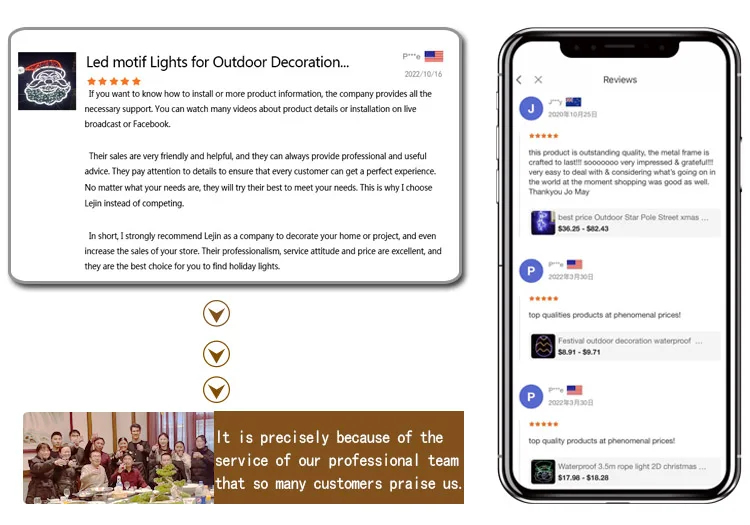**Caption:**

The screenshot from the website displays a detailed review section for "LED Motive Lights for Outdoor Decoration." On the left-hand side, there's an image of a cartoon Santa Claus wearing a red hat, set against a black square background. Below the image are five yellow stars indicating the review rating. Accompanying the image on the left, there's a brief review written in black text, divided into three small sections, with an additional banner positioned at the bottom left. 

On the right-hand side, the website features a cell phone icon displaying three five-star reviews. Each review is associated with a profile picture indicated by initials: "J" for the top review, and "P" for both the middle and bottom reviews. The cell phone icon sports a gray and black outer frame. Above the cell phone, there's an American flag and the date "2022-10-16."

Adjacent to the review section, three brown downward arrows point towards a banner featuring a family gathered around a table on the left. The right side of the banner reads, "It is precisely because of the service of our professional team that so many customers praise us," written in white text on a dark brown background.